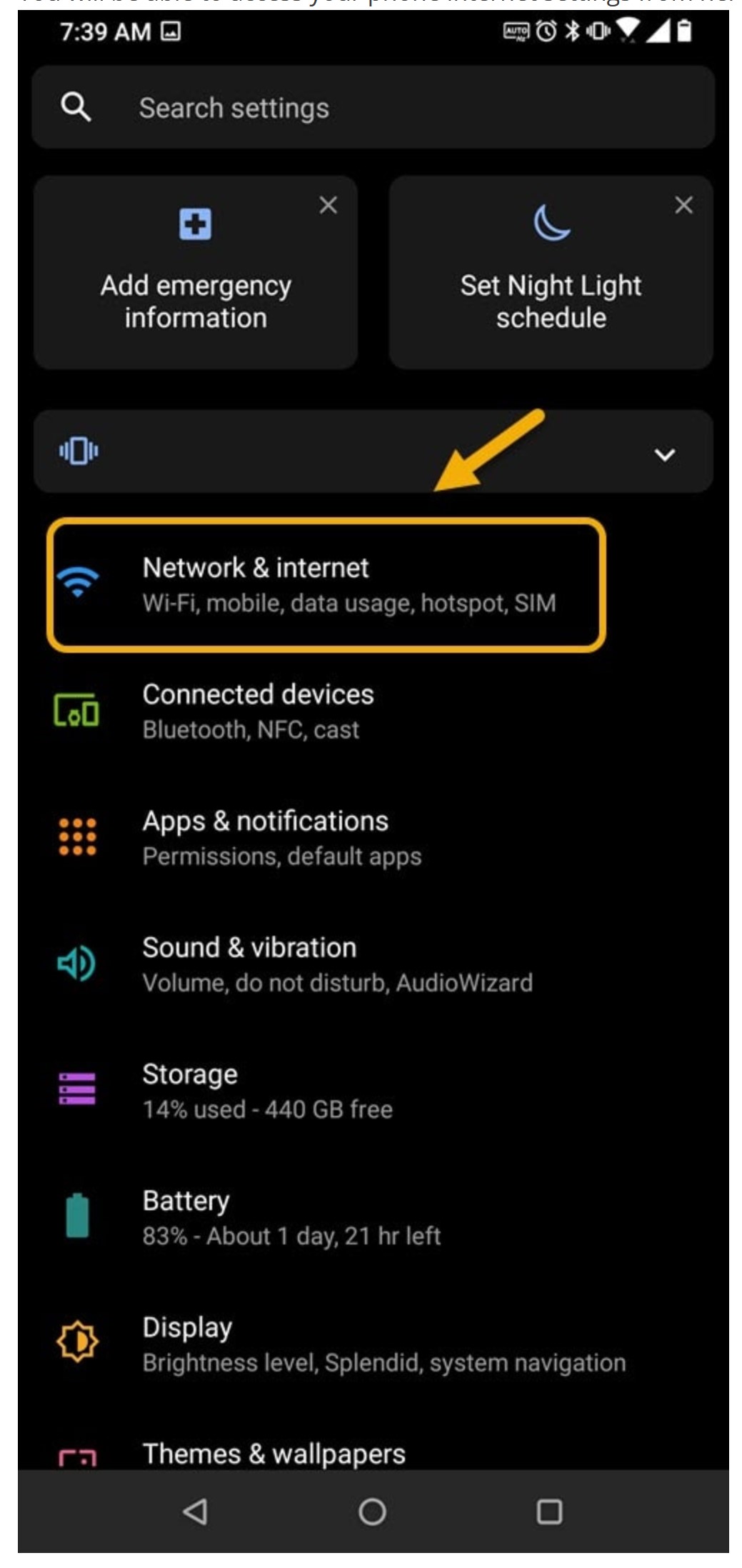Screenshot of an Android phone displaying the settings menu in dark mode. The screen shows a highlighted section with an arrow pointing to the "Network & internet" option, suggesting possible troubleshooting instructions or guidance on how to configure network settings. Underneath "Network & internet," it lists sub-options such as Wi-Fi, mobile data, data usage, hotspot, and SIM. Additional, non-highlighted settings categories are visible, including Connected devices, Apps & notifications, Sound & vibration, Storage, Battery, Display, and Themes & wallpapers. The screen also presents options for adding emergency information and setting up a nightlight schedule. A search bar for settings is available at the top. The status bar at the very top displays icons for battery life, signal strength, and Wi-Fi connection. The background is black, indicating the use of a dark theme.